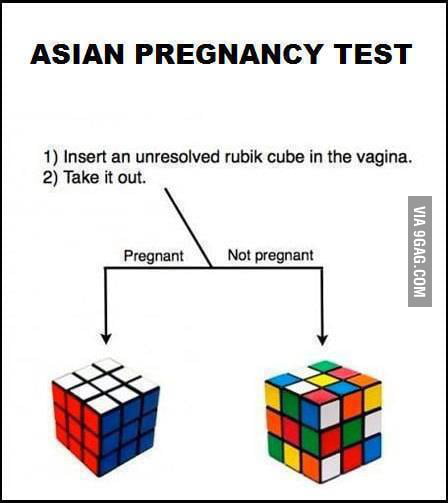The humorous image titled "ASIAN PREGNANCY TEST" displayed against a white background with a black border, outlines a gag test with two steps. Step one instructs to insert an unresolved Rubik's Cube into the vagina. Step two advises to take it out. The subsequent result is depicted with arrows pointing to two different Rubik's Cubes: a solved Rubik's Cube (white on top, red on one side, and blue on another) indicates pregnancy, while an unsolved, multicolored cube (showing various colors like white, yellow, blue, pink, red, and green) signifies not pregnant. The image humorously suggests that the solved Rubik's Cube confirms pregnancy, whereas the mixed-up colors denote no pregnancy. The source of this comedic piece is credited to via9gag.com, printed vertically on the right-hand side.